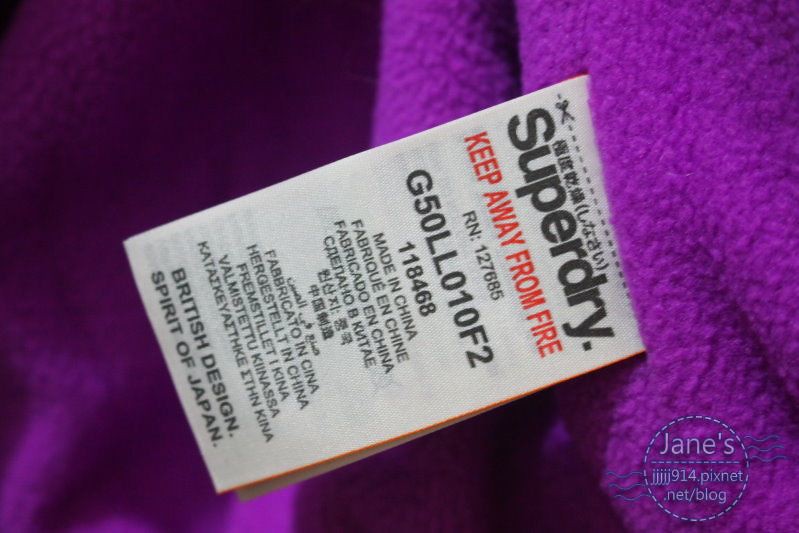This close-up image captures a white clothing tag attached to the fuzzy inside of a purple garment, possibly a sweater or towel. The top of the tag features a pair of scissors and a dotted line indicating where it can be cut. The first line displays "Superdry" in bold black letters, followed by a safety warning in red text reading, "Keep away from fire." Below this, in black text, are the product identifiers: "RN 127685" and "G50 LL01042," followed by "118468." The tag also states "Made in China" and "Fabricado en China," both in English and Spanish, respectively. Multiple translations of "Made in China" follow in approximately eleven different languages. At the tag's bottom, it proudly boasts, "British Design, Spirit of Japan." In the bottom corner, there's a URL for "Jane's," adding a final touch to the detailed label.